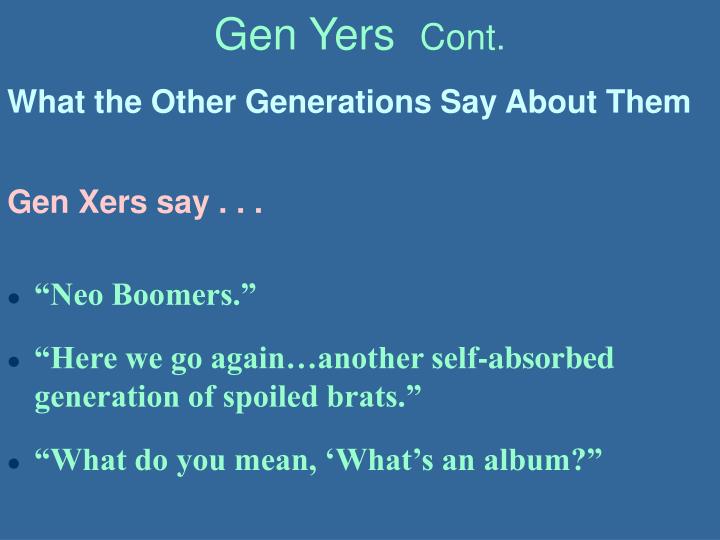The poster features a solid blue background with light green lettering and three pink-highlighted words. At the top, it reads "Gen Years Continued" in lime green text, abbreviated as "Gen Yours, Y-E-R-S. C-O-N-T, period." Below, in white text, it explains, "What the other generations say about them." Highlighted in pink, "Gen Xers say..." introduces a list of three bullet points. Each bullet point is in mint green text and contains a quote: "Neo Boomers," "Here we go again, another self-absorbed generation of spoiled brats," and "What do you mean, what's an album?" The overall design is minimalistic, resembling a presentation slide with no additional graphics.